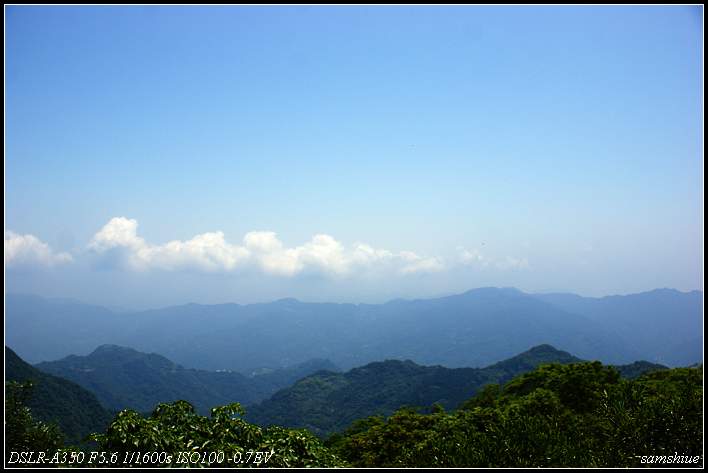The photograph is a detailed landscape captured in full color during daytime. The top third of the image features a clear blue sky, slightly interrupted by a thin layer of clouds stretching from the left side across roughly four-fifths of the image. Below the sky, a distant mountain range with a bluish tint gives a shadowy impression. Closer to the foreground, a darker blue layer of mountains appears. Moving even closer, another small, hillish mountain adds depth to the scene. The immediate foreground reveals a hill covered in green trees. The entire scene is bordered by a black frame. 

In the bottom left corner, white text reads "DSLR A350 F 5.6 1/1600 ISO 100 -0.7 EV," while the bottom right corner shows another small white text that reads "Samchui." The overall composition beautifully juxtaposes the varying blue hues of the mountains with the lush greenery, under an expanse of clear sky and sparse clouds.